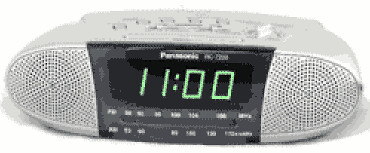The image depicts a somewhat contemporary yet old-fashioned-style digital clock radio, possibly a Panasonic, in a blurry photograph or computer-generated rendering. The clock radio is white but appears grayish due to the varying shades of lighting in the photo. It features a rectangular shape with rounded edges, equipped with numerous buttons and dials on the top for setting the alarm, tuning the radio, and adjusting the time. The central section of the front displays the time reading "11 o'clock" in a green digital format on a black screen. Surrounding the clock face are circular speaker covers with tiny perforations. The radio dial and the FM/AM indicators below the clock display are visible but not legible due to the image's blurriness. The device casts a shadow against an otherwise white background where the surface context has been cut out, focusing the view on the clock radio itself.